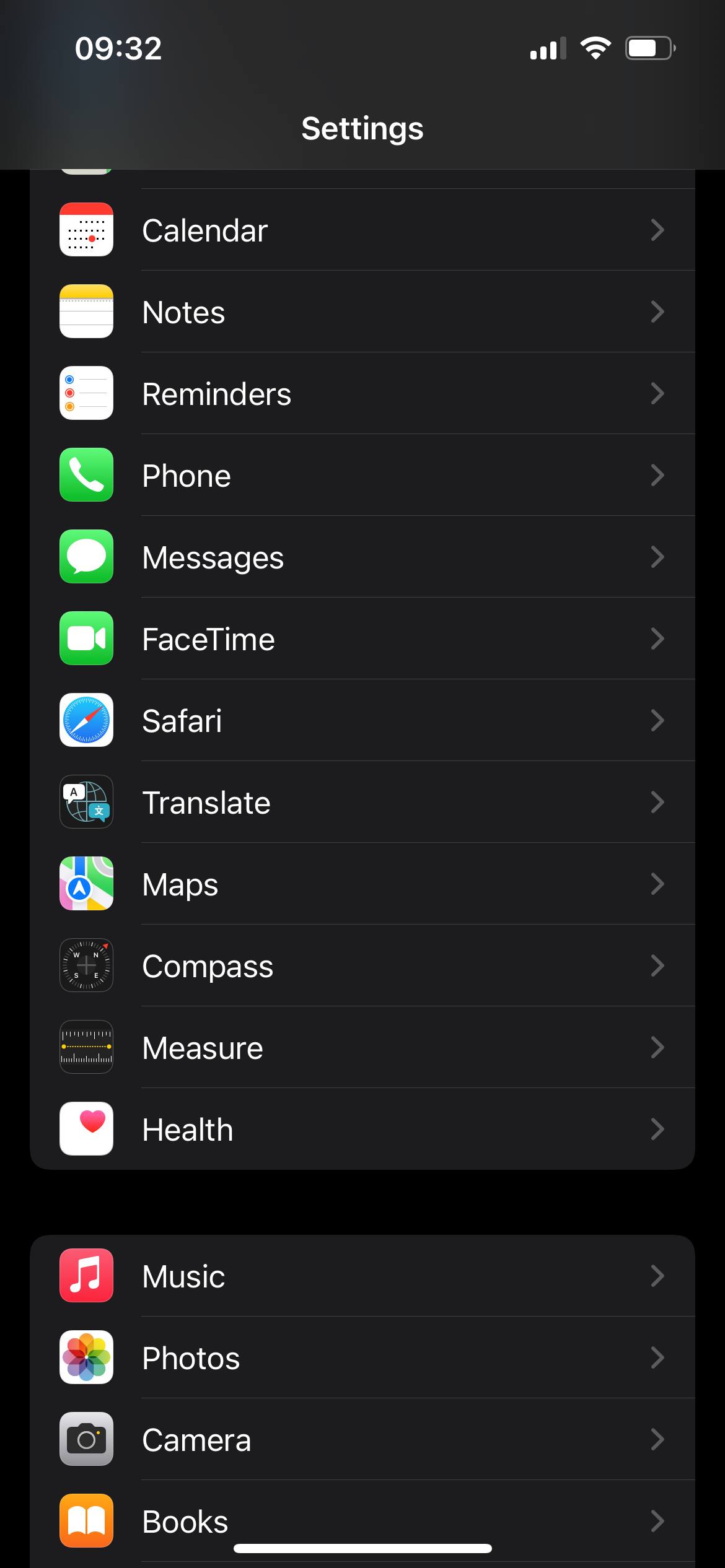The image depicts a smartphone’s settings page with a black background. At the top, the time is displayed as 9:32, alongside various indicators including cellular signal bars, Wi-Fi status, and battery level. Below, the word “Settings” is prominently featured in white text.

The settings options are listed with corresponding icons:

1. **Calendar**: Represented by a red and white calendar icon.
2. **Notes**: Illustrated with a yellow and white notepad icon.
3. **Reminders**: Depicted with a white icon featuring colorful check-off circles in blue, red, and yellow.
4. **Phone**: Shown with a green background and a white phone icon.
5. **Messages**: Displayed with a green background and a white speech bubble icon.
6. **FaceTime**: Marked by a green background with a white video camera icon.
7. **Safari**: Illustrated with a blue circle and a red and white compass pointer.
8. **Translate**: Represented by a globe icon featuring an "A" and another language character.
9. **Maps**: Depicted with an icon resembling a map and a blue location marker.
10. **Compass**: Shown with a black background displaying the cardinal directions (north, south, east, west).
11. **Measure**: Represented by an icon of a tape measure.
12. **Health**: Illustrated with a white background and a pink heart icon.
13. **Music**: Depicted with a red background and a white musical note icon.
14. **Photos**: Shown with a colorful circular icon, featuring shades of purple, orange, green, and blue.
15. **Camera**: Represented by a traditional camera icon.
16. **Books**: Illustrated with an open book icon on a brown background.

The overall interface is simple yet visually organized, allowing easy navigation through various settings options.